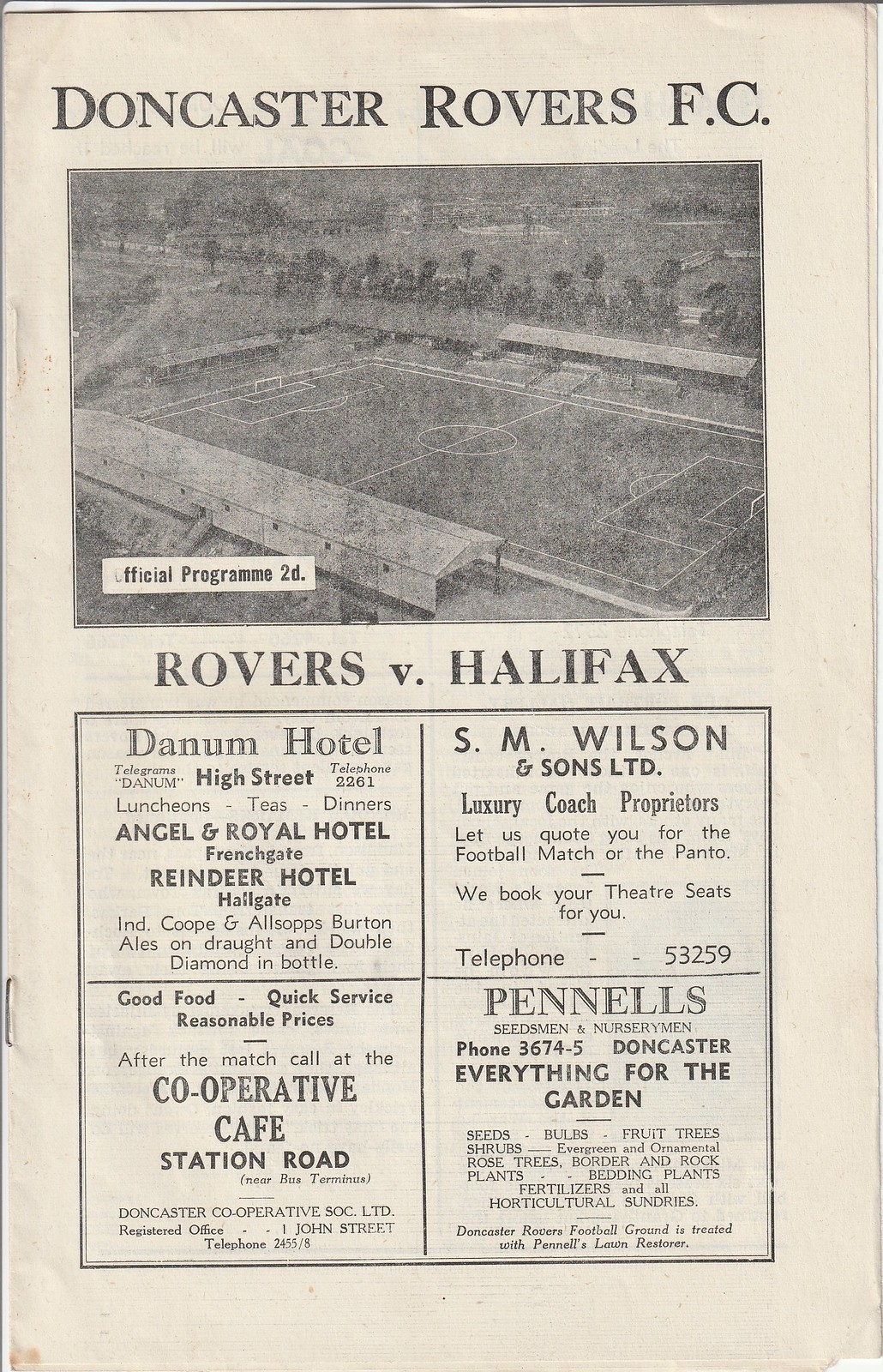This is an aged advertisement page from an old newspaper or magazine, presenting a vintage soccer theme focused on Doncaster Rovers F.C. It features an official program note "2D" in black and white. The top of the page prominently displays "Doncaster Rovers F.C." alongside an image of a soccer field. Below, it details a match between "Rovers vs. Halifax." The lower portion of the page is methodically divided into a series of four squared advertisements promoting various local businesses. The top left square highlights the Danum Hotel on High Street offering luncheons, teas, and dinners. Adjacent to that, on the top right, is an advertisement for S&M Wilson & Sons LTD, a luxury coach provider, complete with a contact phone number. The bottom left features the Cooperative Cafe on Station Road boasting good food, quick service, and reasonable prices, encouraging patrons to visit after the match. Finally, the bottom right square promotes Pennell's, Seedsmen & Nurserymen, with a focus on gardening supplies, also providing a contact number. All elements are rendered in the black, gray, and white tones typical of the period, enhancing the historical ambiance of the piece.